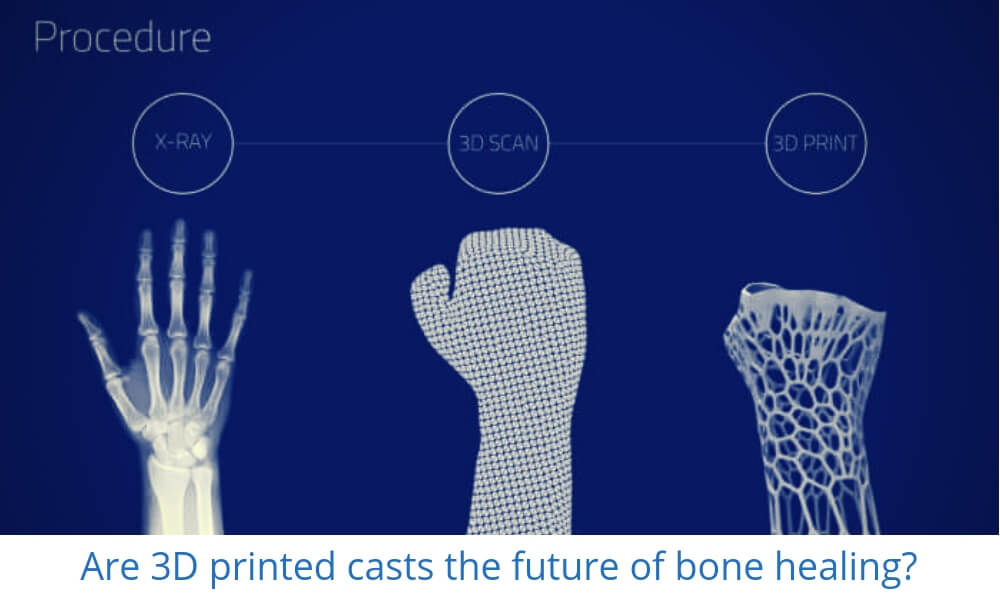In this scientifically themed image, a streamlined timeline of a medical procedure is depicted against a dark blue background with white text. At the top left corner, the word "Procedure" is prominently displayed. The timeline is divided into three sections, each illustrating a different step of the process involving 3D technology for bone healing. 

The first section, labeled "X-ray," showcases an x-ray image of a skeleton hand, highlighted with bright white light. A line connects this to the second section, labeled "3D Scan." Here, the image portrays a digital scan of the hand, which appears to be missing fingers and looks as though it is holding a glove. This scan has a net-like appearance with parts of the thumb and fingers missing or semi-transparent. 

The final section, labeled "3D Print," displays a 3D printed model of the arm, characterized by its white color and circular holes. Unlike the previous images, this one seemingly lacks details of the hand, emphasizing the technological transformation from scan to printed cast.

Beneath the entire timeline, a thought-provoking question in blue text aligns perfectly with the image's theme: "Are 3D printed casts the future of bone healing?" With its minimalist design and clear blue and white color scheme, the image effectively communicates the progressive steps involved in creating 3D printed casts for medical purposes.